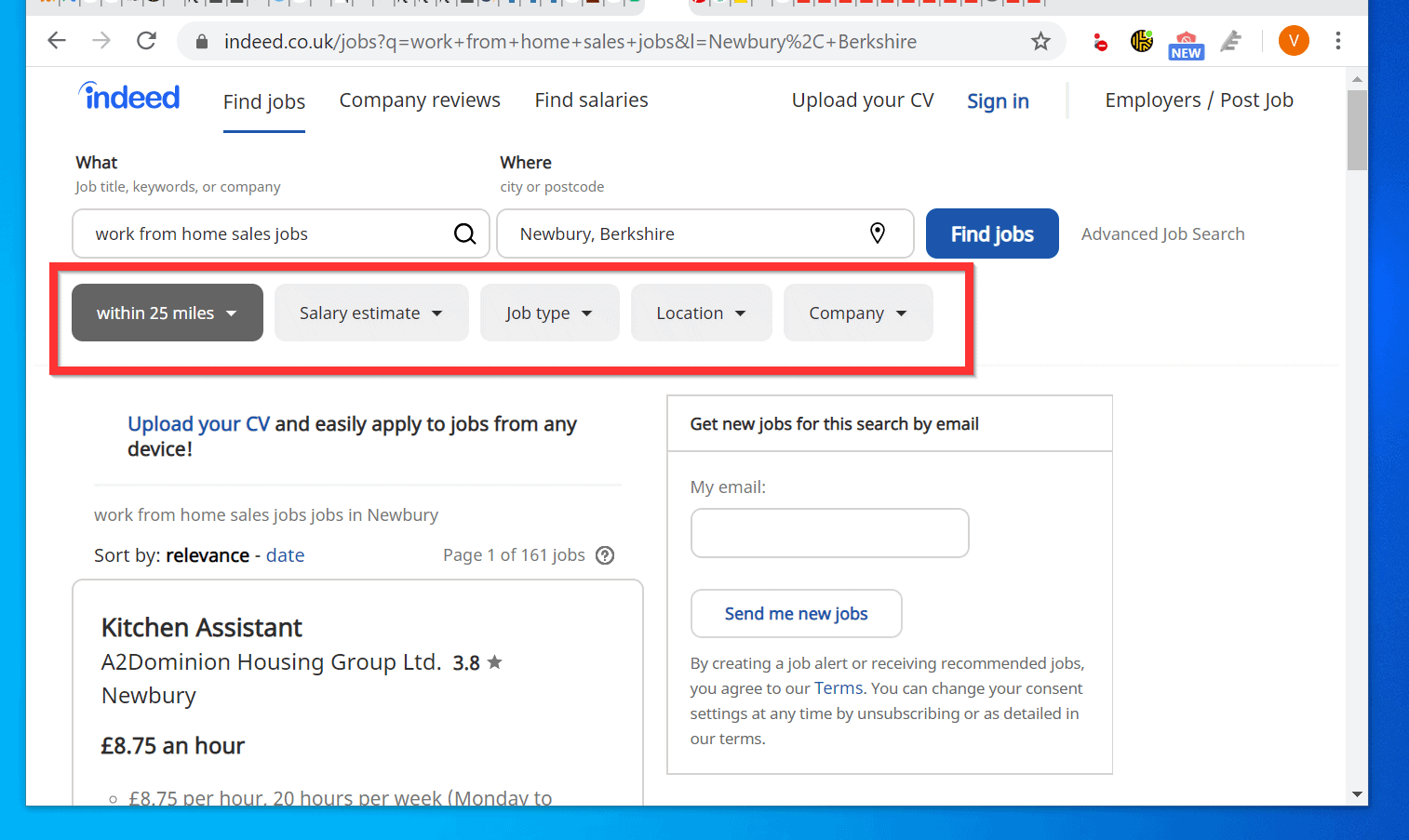The image is a screenshot from the Indeed website, specifically from the UK domain (indeed.co.uk/jobs), where a user is conducting a job search. Although the top of the screen is cropped, the top left corner prominently displays the Indeed logo in blue. 

The URL at the top highlights the search path, indicating a job search in progress. Several navigational categories are visible: "Find jobs," "Company reviews," "Find salaries," "Upload your CV," "Sign in," and a section for employers to post jobs. The "Find jobs" category is currently selected, evidenced by its underline, and it showcases the search bars for job queries.

The search interface includes two primary fields: "What" and "Where." The "What" search bar is intended for entering job titles, keywords, or company names, while the "Where" search bar is designated for cities or postcodes. In this instance, the user has entered "work from home sales jobs" in the "What" field and "Newbury, Berkshire" in the "Where" field. Next to these fields is a blue button with white text that reads "Find jobs."

Below the search bars, there are additional sorting options, encased in a bold red outline for emphasis. The highlighted sorting category is "Distance," set to within 25 miles. Other available sorting categories include "Salary estimate," "Job type," "Location," and "Company," though none of these have been selected yet by the user.

Overall, the screenshot provides a detailed overview of a job search for remote sales positions within a 25-mile radius of Newbury, Berkshire, on the Indeed UK website.